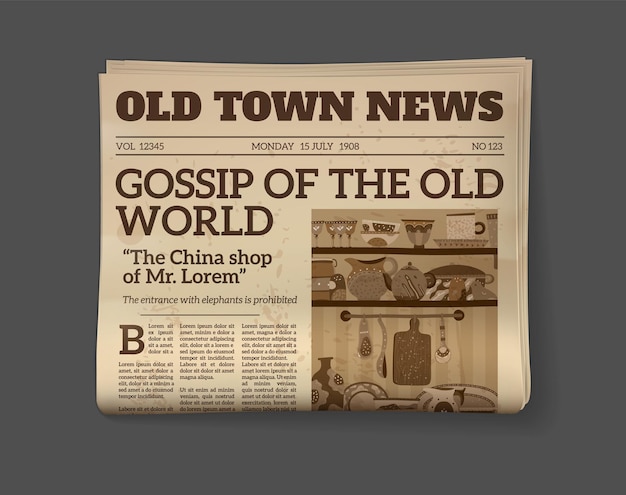In the image, we see a vintage cover of a folded newspaper titled "Old Town News," prominently displayed against a dark gray background. The newspaper, thick and suggesting the feel of old-style publications, is from Volume 12345 and dated Monday, 15 July 1908, Number 123. The headline reads, "Gossip of the Old World," with a subtitle in quotes, "The China Shop of Mr. Lorem." Below the title, an article begins with "The entrance with elephants is prohibited." On the left side, three columns of text mark the start of the article. To the right, there is an illustration in shades of brown, tan, and white depicting shelves filled with kitchen utensils—mugs, bowls, dishes, a serving pot, a teapot, and a large ladle hanging from a rack. The scene looks like the interior of a kitchen or shop, complementing the subheadline of the newspaper.